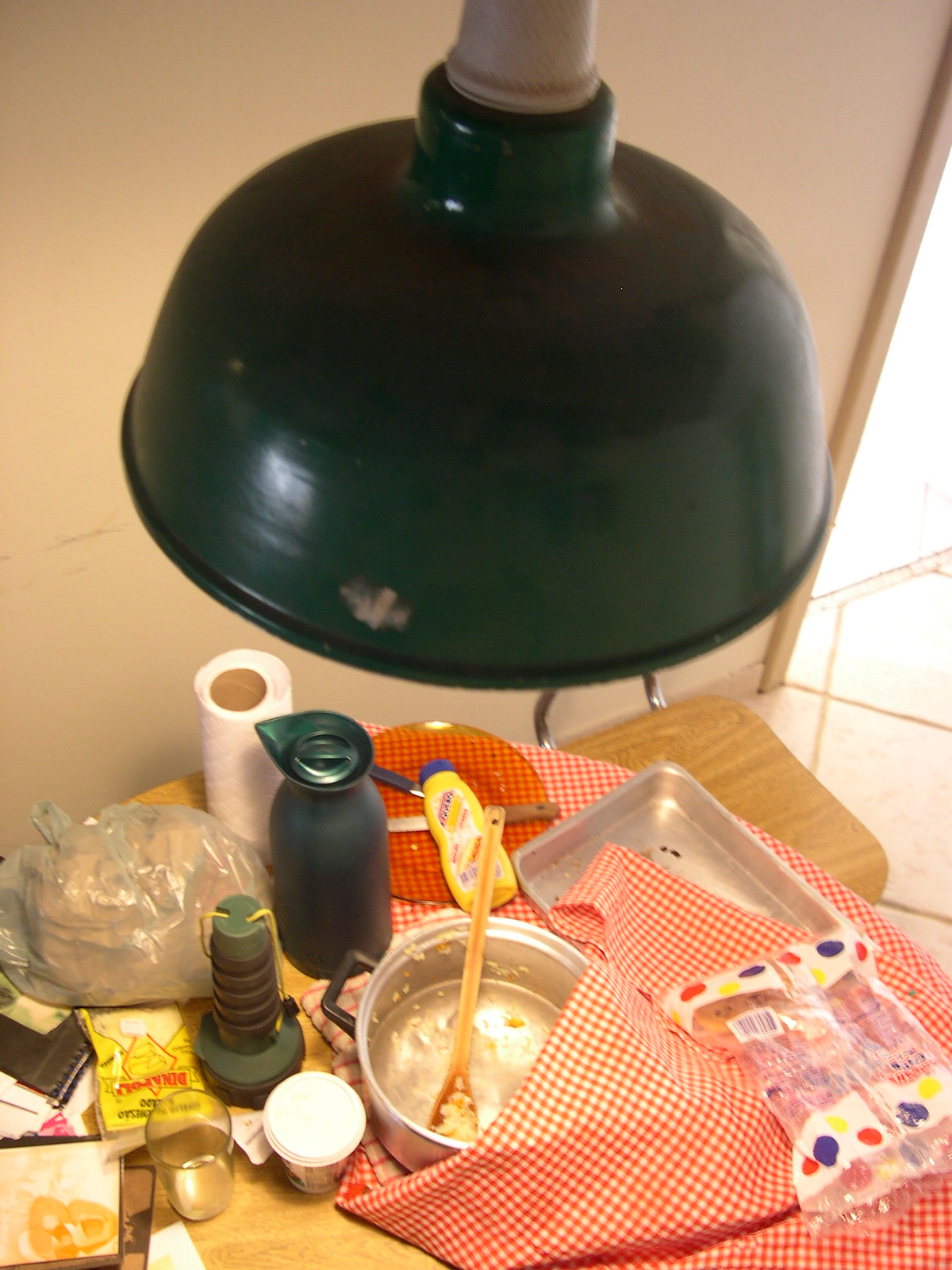A messy kitchen counter illuminated by a hanging ceiling light showcases a chaotic yet lived-in scene. At the center, a kitchen table draped with a red and white checked tablecloth catches the eye. On the table, a saucepan with food debris clings to a wooden spoon, suggesting a recent meal, possibly rice. Nearby, another pan shows clear signs of use with visible stains. A squeeze bottle of butter adds to the clutter, along with an orange plastic plate holding a knife and another utensil. A roll of paper towels and an empty plastic bag, likely once containing white bread, contribute to the disarray. Various other objects are scattered around, completing the picture of a busy, unkempt kitchen environment.